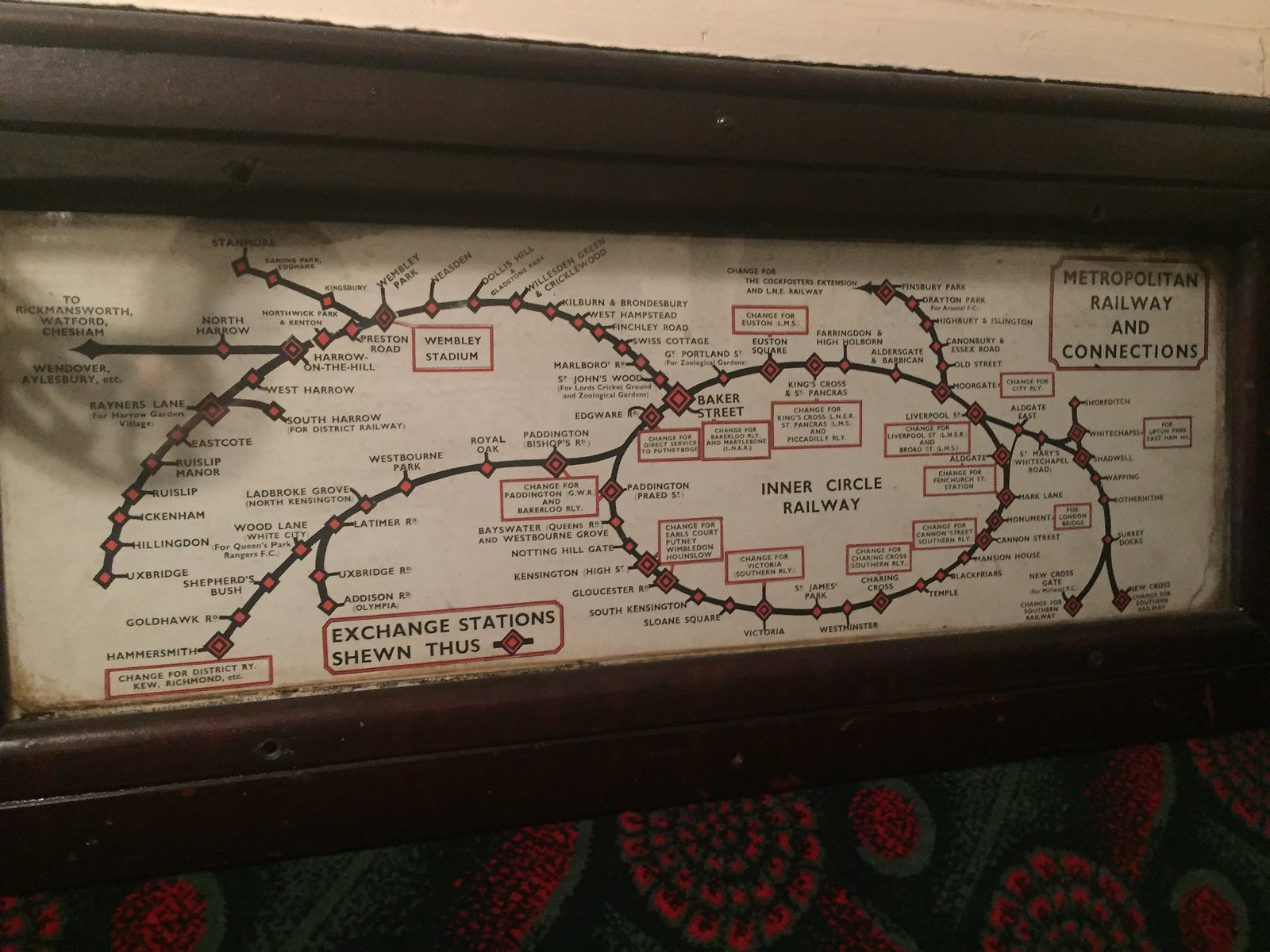The image showcases a historical map titled "Metropolitan Railway and Connections," encased in a sturdy wooden frame with a rich brown top and bottom. The white card inside depicts a detailed illustration of railway routes, characterized by red dots indicating stops and exchange stations, and features a notable circular route referred to as the Inner Circle Railway. This map seems to be a representation of London's transit system, highlighting stops such as Preston Road with a line extending to Wembley Stadium. The frame extends slightly off the left edge of the image, while the right side reveals a patterned green and red wallpaper beneath the encasement, suggesting an indoor setting. The upper right-hand corner of the map bears the title, and the entire setup, encased behind glass with a visible keyhole mechanism, appears notably vintage, resting against a tan wall.